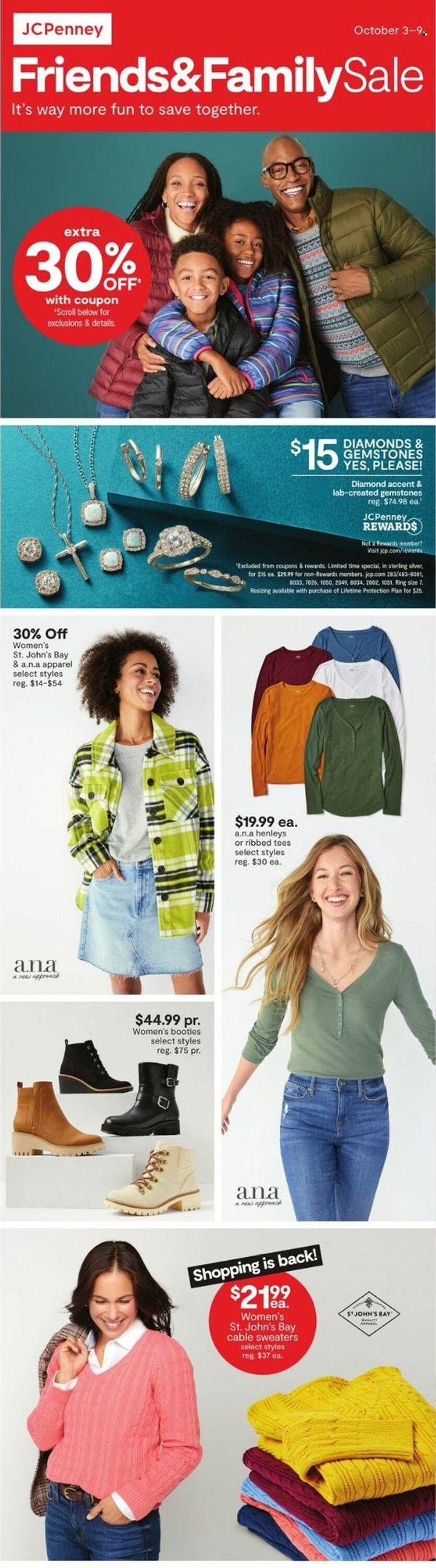This advertisement from JCPenney features a Friends and Family Sale lasting from October 3rd through October 9th, prominently displayed in a tall, narrow format. The top section of the ad has a bold red block with white text that reads "JCPenney Friends and Family Sale, October 3rd through the 9th. It's way more fun to save together." Immediately below, a photograph showcases a happy family embracing, set against a dark green backdrop, with a circular badge highlighting an "Extra 30% Off with Coupon."

Moving down, the next section displays a collection of jewelry alongside a promotional message. Below the jewelry, three distinct images are featured: 
- On the left, a woman in a colorful jacket and jean skirt is turned to her left, accompanied by an advertisement for the clothing.
- In the center, an ad for women's boots is delicately placed between the images.
- On the right, another woman faces forward, wearing a green shirt and blue jeans, alongside an advertisement for the shirts.

The bottom part of the ad includes a woman looking down and forward, dressed in a cozy sweater, with an array of sweaters displayed next to her. The accompanying text enthusiastically declares that "Shopping is Back."

These images, excluding the jewelry section, are set against a muted gray background, emphasizing the range of apparel and accessories available during the sale.